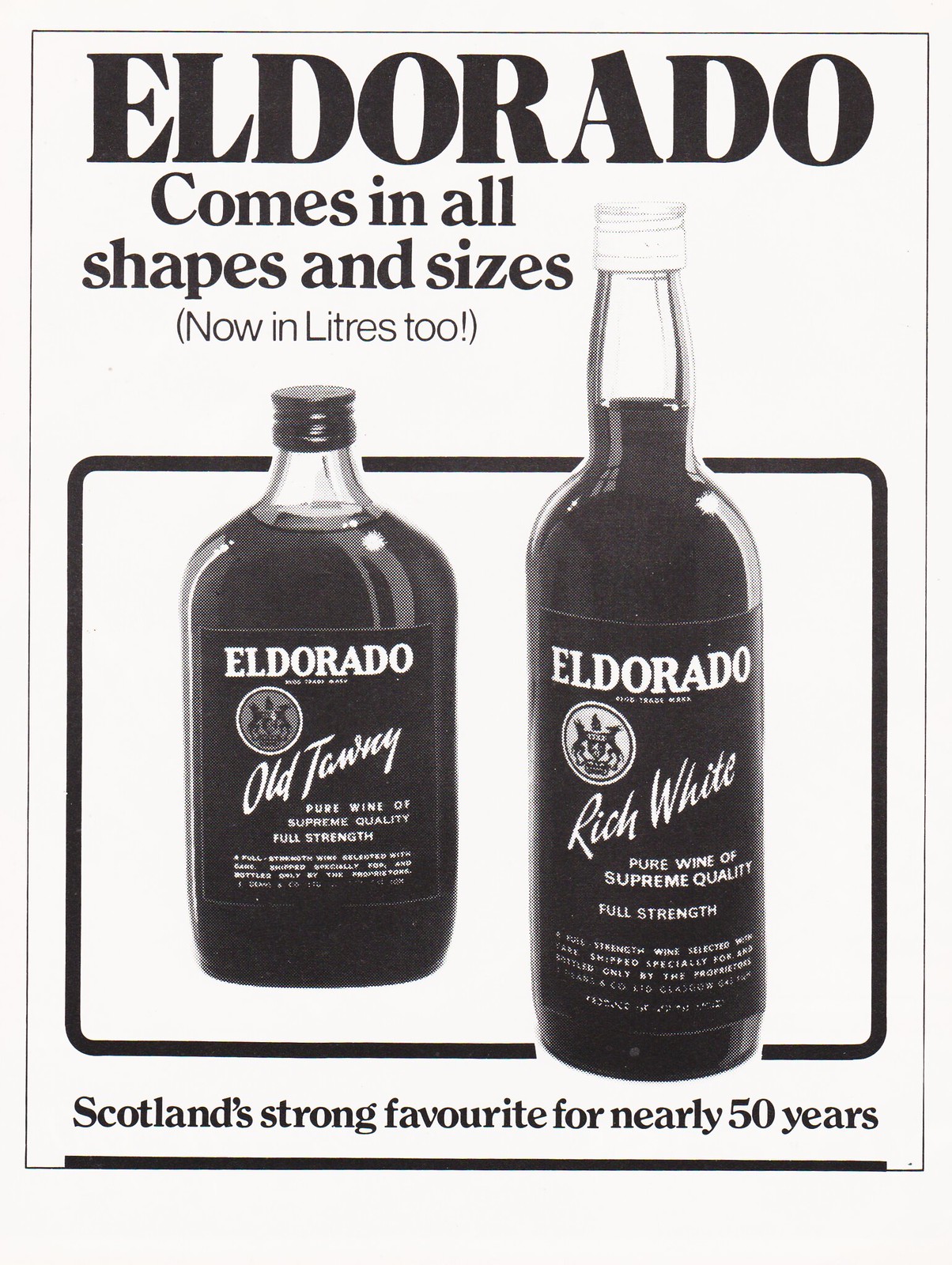The black-and-white poster advertises Eldorado, a Scottish wine, prominently displaying its name at the top in bold, capital letters. Beneath, a phrase announces "comes in all shapes and sizes" with a note in parentheses stating “now in liters too!” Centered in the middle of the poster, two bottles of Eldorado are depicted within a rounded rectangle. On the left, a smaller, flask-sized bottle labeled "Eldorado Old Tawny" features a black screw cap and a crest with two griffins. To the right, a taller, traditional wine bottle labeled "Eldorado Rich White" boasts italicized text and a white screw cap, with smaller print beneath reading "Pure Wine of Supreme Quality." At the bottom of the poster, bolded text proclaims, "Scotland's Strong Favorite for nearly 50 years." The entire design, including the bottle images and liquid inside, is rendered in black and white.